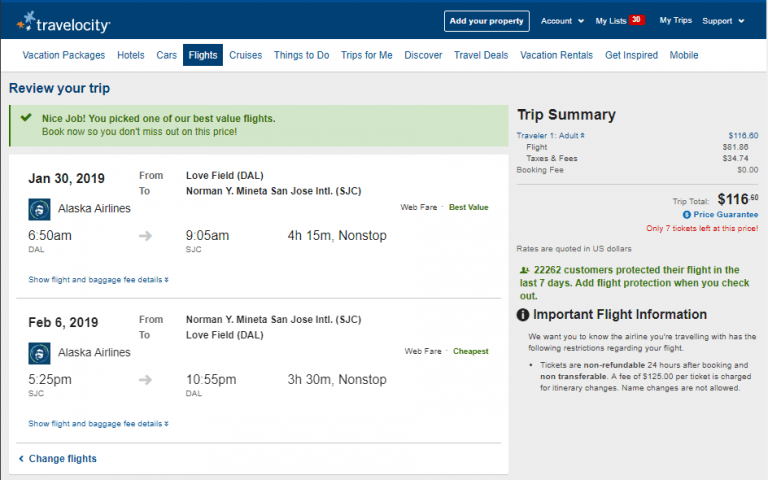Here is the cleaned-up and detailed caption for the image:

---

This is a detailed screenshot of a webpage from the travel booking site, Travelocity. The page features a web interface set against a dark blue background with white text on the top navigation bar. The topmost section includes options like "Add Your Property," "Account," "My List" (indicating there are 30 items in the list), "My Trips," and "Support" with a pull-down context menu.

Below the navigation bar, a secondary menu on a white background displays categories such as "Vacation Packages," "Hotels," "Cars," "Flights" (which is currently highlighted in black to indicate selection), "Cruises," "Things to Do," "Trips for Me," "Discover," "Travel Deals," "Vacation Rentals," "Get Me Inspired," and "Mobile."

The main content of the page shows a summary of a selected trip, confirming the user has picked an optimal value flight. The highlighted text states, "Nice job, you picked one of the best value flights!" followed by a green check symbol. The trip details specify the following:

- **Departure:** January 30th, 2019, from Love Field, Dallas to Norman Y. Mineta San Jose International Airport (SJC) via Alaska Airlines. Departure is at 6:50 AM, with arrival at 9:50 AM, totaling a 4-hour and 15-minute non-stop flight.
- **Return:** February 6th, 2019, from Norman Y. Mineta San Jose International Airport back to the original destination via Alaska Airlines. Departure is at 5:25 PM, with arrival at 11:55 PM, totaling a 3-hour and 30-minute non-stop flight.

A summary at the page's footer outlines the total cost:

- **Flight fee:** $81.00
- **Travel fee:** $34.74
- **Booking fee:** $0.00
- **Total cost:** $116.00

The summary also mentions a limited availability with only seven tickets left for this particular flight, accompanied by a "Price Guarantee" note. Additionally, there are various legal disclaimers and policy details listed below the summary.

---